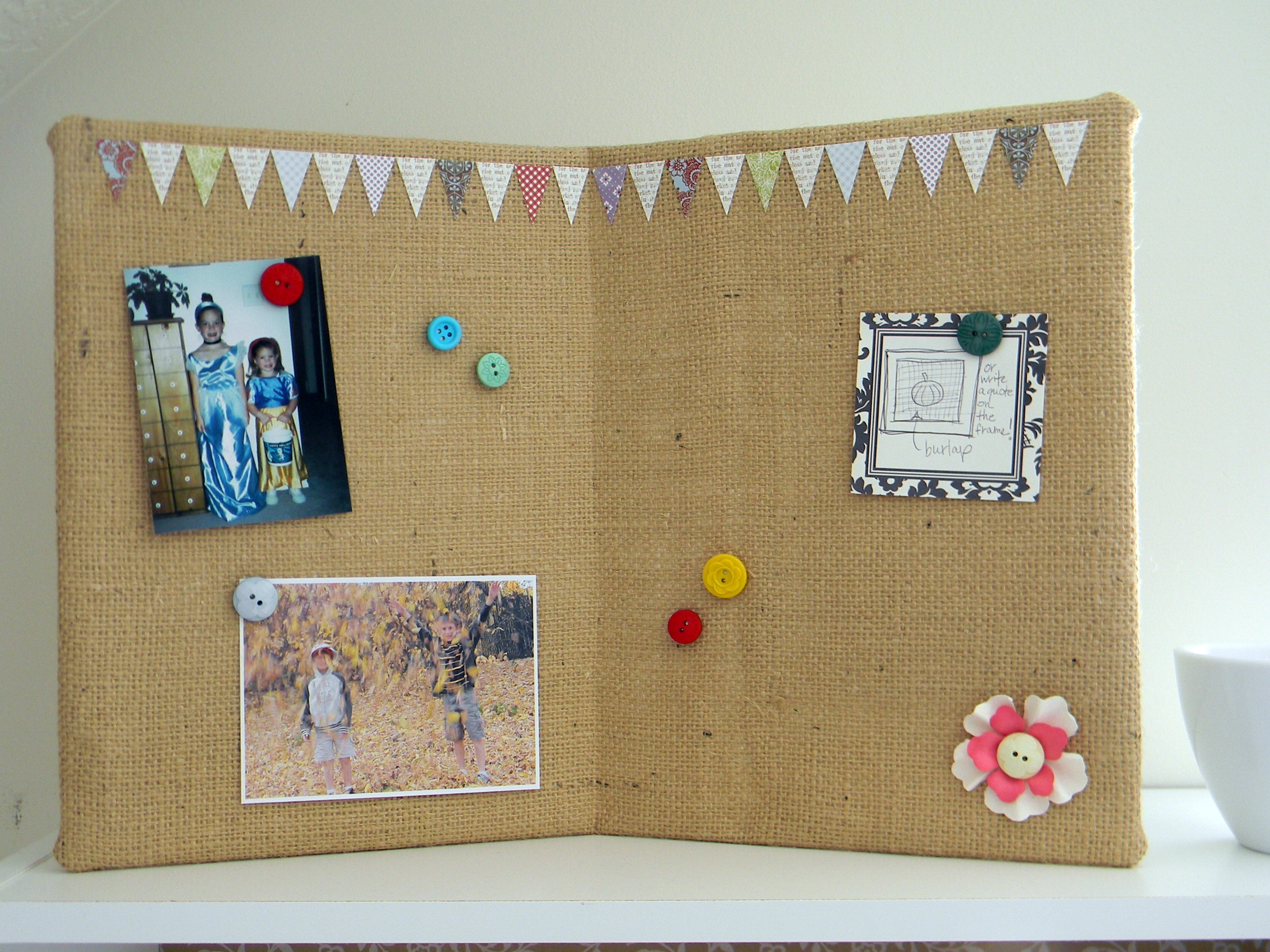This image depicts a homemade burlap bulletin board, positioned at a slight angle on a white shelf against an off-white wall. The board, reminiscent of a folded book, is covered in tan-colored burlap cloth. At the top, colorful miniature pennant flags add a playful touch. Several photos adorn the board, including a picture of two little girls in elaborate dresses, possibly princess costumes, and another photo of two children playing in a leafy field. These images are secured by decorative push pins resembling buttons in various colors. Additionally, there is a hand-drawn picture and a diagram or list on the right side. In the bottom right corner, a pink flower with a cream-colored button center completes the display. Next to this bulletin board, a white porcelain or crock bowl adds a subtle accent to the overall arrangement.